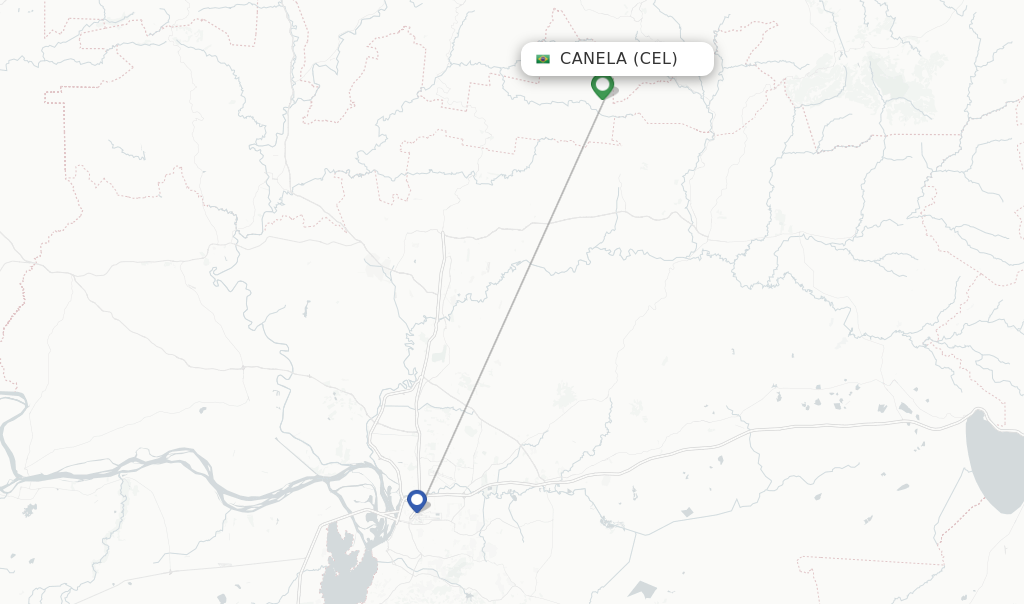The image is an overhead view of a map depicting Central and South America with a solid white outline contrasted against a very gray background. Above South America and to the east of Central America, Cuba is visible. There is a line that starts somewhere in South America, crosses through Brazil, and appears to extend northwards, potentially ending in Florida. The map includes some text at the top written in black with a white border, though it's partially cut off and unreadable. The line traversing the map covers a significant distance, but its exact purpose or representation remains unclear.